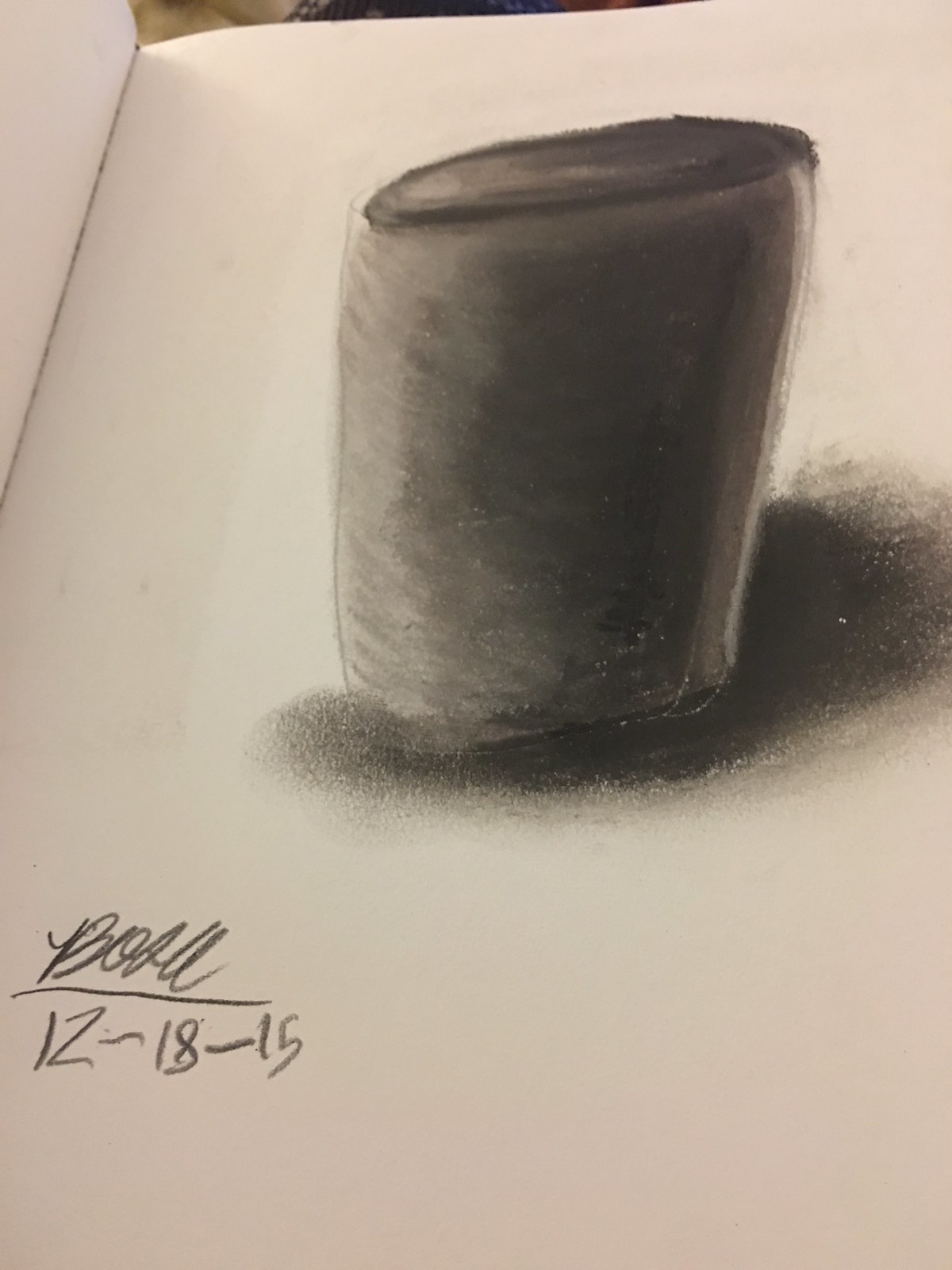This is a detailed charcoal drawing displayed on a drawing pad, clearly visible against a background that reveals part of the table in the upper left and middle top sections of the image. The central subject of the drawing is a cylindrical object with a pronounced rim at the top. A light source is positioned on the left, casting significant shadows that enhance the cylinder's three-dimensional appearance. Notably, preliminary sketch lines are faintly visible on the left side of the cylinder. The right side of the cylinder features intense shadowing, interrupted by a stark white line that runs vertically. This heavy shadowing extends to the bottom right corner of the object, emphasizing the depth and contrast in the artwork. In the lower left corner of the drawing, the artist's signature appears in cursive, reading "B-O-S-A" with a line underneath it, dated 12-18-15.